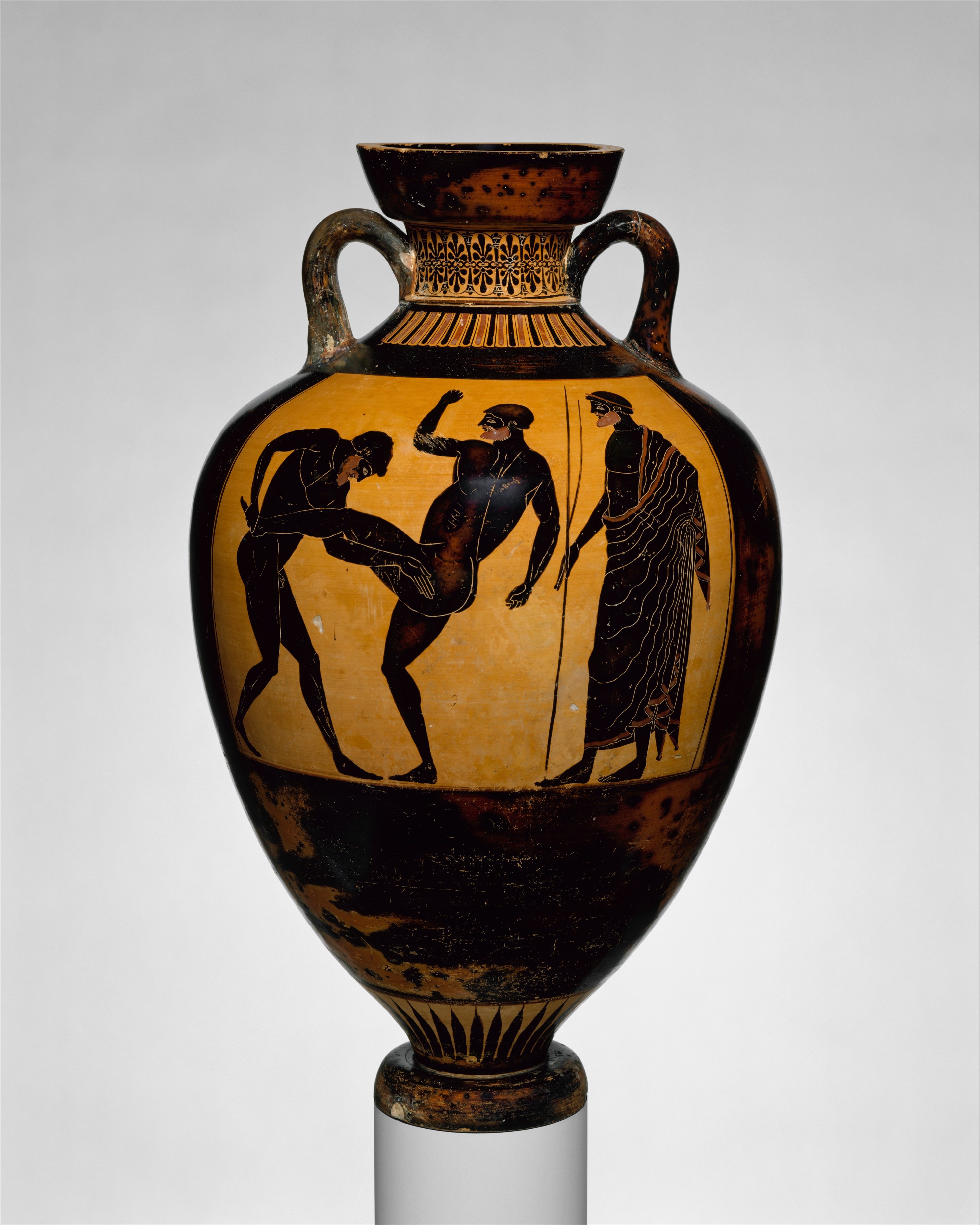This image features a detailed ancient vase, believed to be of Greek origin, displayed on a white pedestal against a gray-white background. The vase, primarily of a deep, reddish-brown color with lighter brown and dark brown areas, is made of glass or possibly inlaid wood with a sophisticated design. It has a wide body with two handles near the top and an ornate opening resembling a cup. 

The top section of the vase is adorned with gold designs, including small crosses and bars, adding a rich, luxurious feel. Below this, a vivid scene is depicted: set against a yellow background, three figures engage in what seems to be a historical or mythological event. The central figure, shown in dynamic motion, is kicking another figure who is doubled over in apparent pain. Both are wearing dark blue garments with orange accents. Observing them is a third figure dressed in a long, blue robe with orange stripes, holding a staff that splits into two points, resembling a pitchfork. 

Intricate orange patterns intersperse the lower sections, transitioning into a dark brown base designed to look like little gold goblets leading to a sturdy foundation. This vase, with its rich historical imagery and detailed craftsmanship, gives a glimpse into a past civilization's artistry and storytelling.